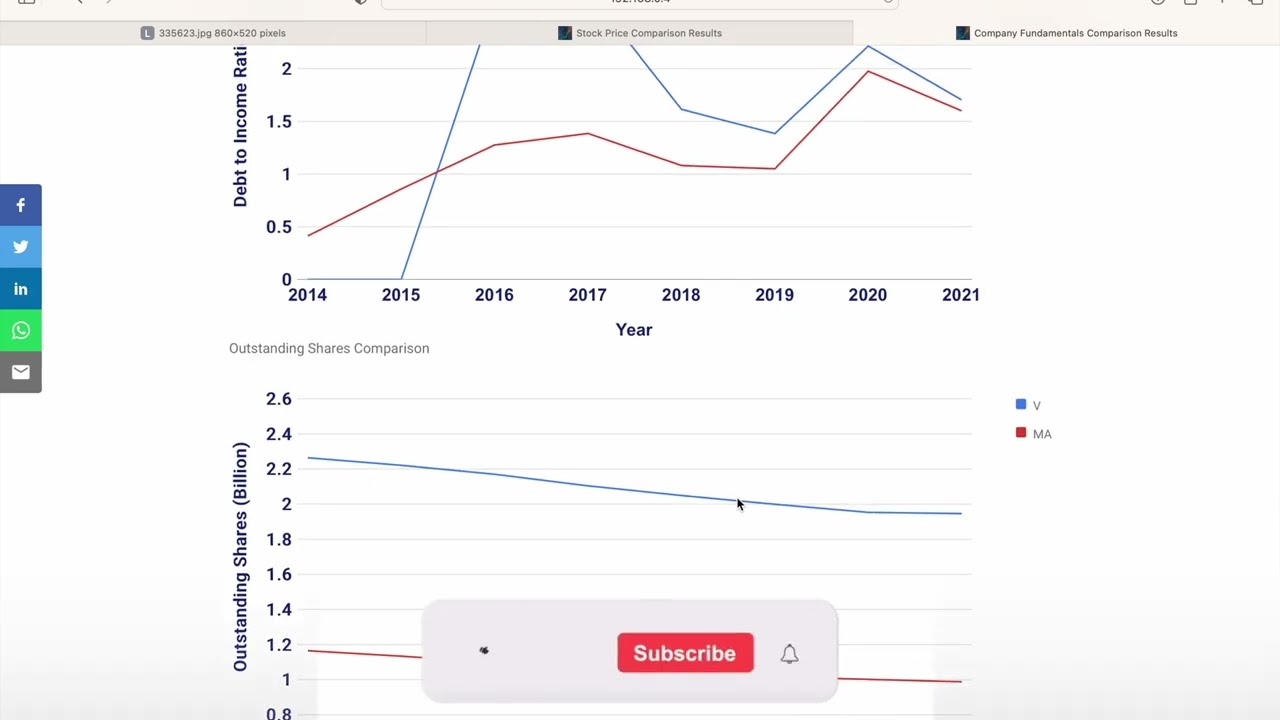The image appears to be a screenshot of a computer screen, possibly an Apple device, featuring two line graphs. On the far left side of the screen, there are icons for social media and communication platforms: a blue Facebook "F", a white Twitter bird, a LinkedIn "IN", a WhatsApp speech bubble with a phone, and an envelope symbolizing email. 

The top graph is labeled "Debt-to-Income Ratio," with the horizontal axis showing years from 2014 to 2021. The vertical axis partially displays the term "debt to income ratio." In this graph, a red line zigzags across the years, while a blue line crosses above it and runs parallel toward the right side. 

The bottom graph is labeled "Outstanding Shares" with the vertical axis indicating "Outstanding Shares (Billion)" in black text. The visible part of the graph shows values scaling from 0.8 up to 2.6 billion. Similar to the top graph, this one also features red and blue lines, with both lines trending diagonally. 

At the bottom of the image, there is a rectangular box containing a dark red subscription button featuring white letters that say "subscribe," likely accompanied by a bell icon. The overall impression is of financial data being reviewed, possibly for a presentation or analytical purposes, with social media and communication icons suggesting sharing or discussing the information online.